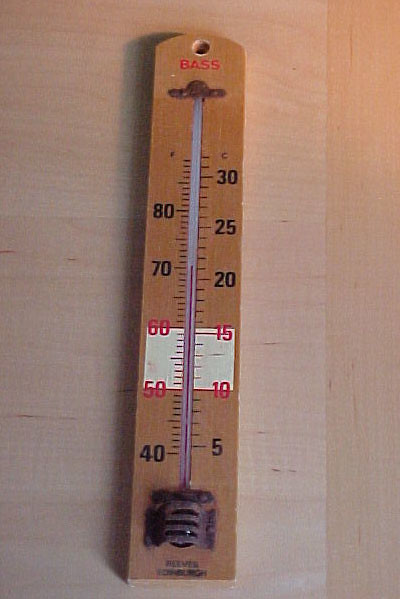The image captures a vintage, rectangular thermometer with a rich, dark brown color, positioned vertically. The background is a light tan, possibly wooden wall, showcasing subtle grain patterns. The wall features a corner near the right-hand edge. The thermometer narrows as it ascends and concludes with a rounded, semi-circular top, where a hole for mounting is visible. Prominently displayed in red letters at the top is the word "BASS.” Below it, there’s a space for a screw, ensuring stable installation.

The central section of the thermometer consists of a clear, whitish meter containing red mercury, securely held at the base by a black metallic component. The left side of the mercury column features numerical markings ranging from 40 to 80, with a highlighted red section denoting the 50 to 60 range. Conversely, the right side scales from 5 to 30, with a similar red-highlighted section between 10 and 15. Toward the bottom, there is faded, difficult-to-read black lettering, indicative of the thermometer’s age and usage.